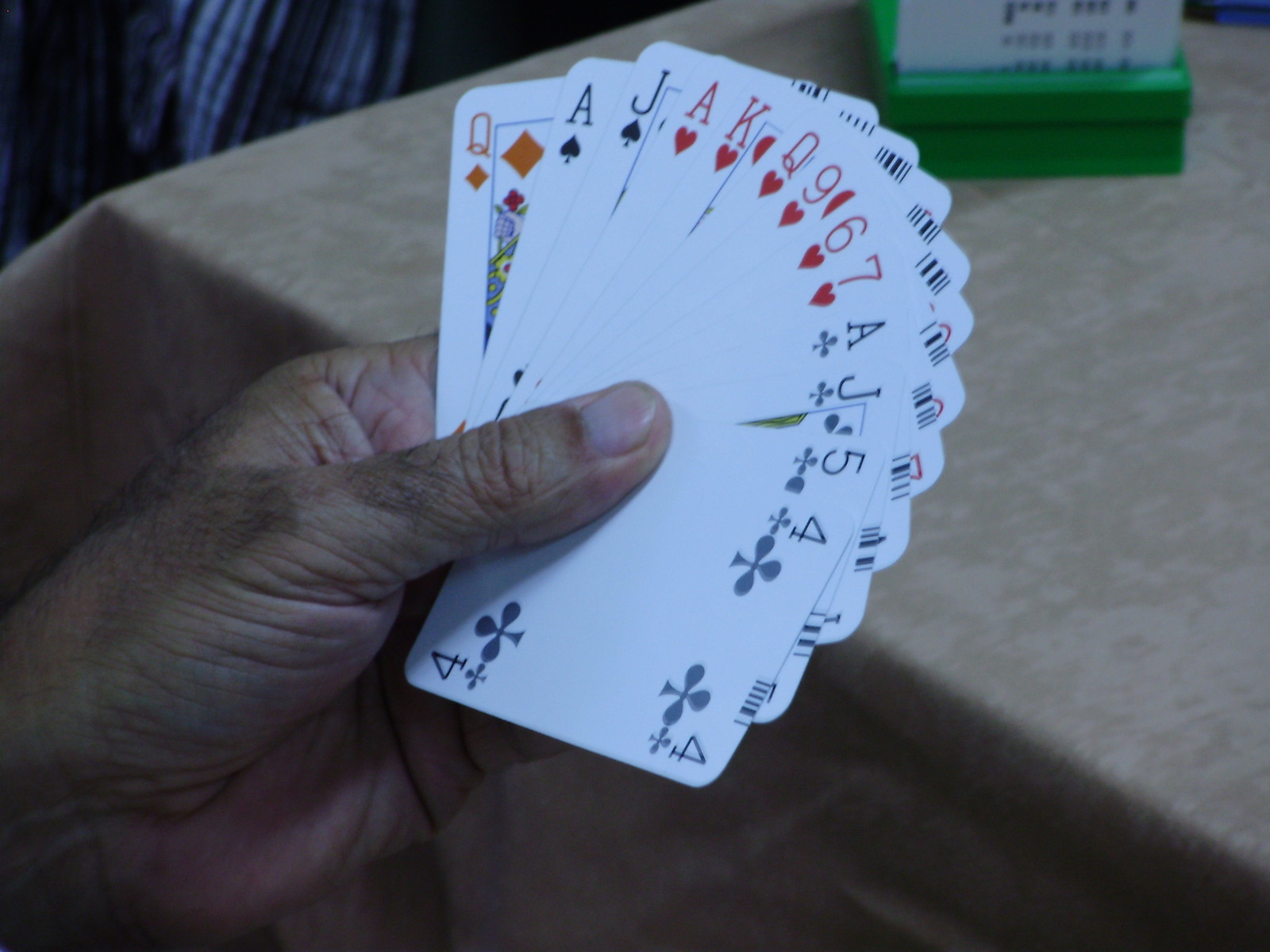The image features a wrinkled hand, likely belonging to an older person, extending from the left and holding a spread of playing cards. The cards are arranged by suit and color, starting from the left with a Queen of Diamonds, followed by an Ace of Spades, Jack of Spades, Ace of Hearts, King of Hearts, Queen of Hearts, 9 of Hearts, 6 of Hearts, 7 of Hearts, Ace of Clubs, Jack of Clubs, 5 of Clubs, and 4 of Clubs. The background includes a beige tabletop, possibly with a place mat, a green box with white sides featuring unreadable text, and a blue fabric object in the top left corner whose purpose is unclear.